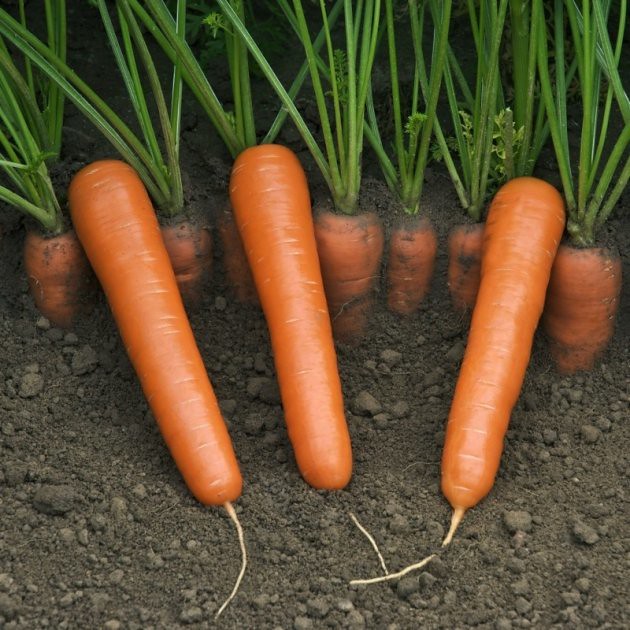In this vibrant garden photograph, three freshly harvested carrots with their roots intact lie in the foreground, while a row of at least seven half-buried carrots, still sporting their bright green stems, can be seen behind them. The harvested carrots, now stripped of their greenery, have a glossy shine, suggesting they've been cleaned, adding to their vivid orange hue. The soil has a soft, grayish-brown appearance, creating a rich contrast with the carrots. Though we can't see the sky, the scene appears sunlit, emphasizing the carrots' freshness and vitality.